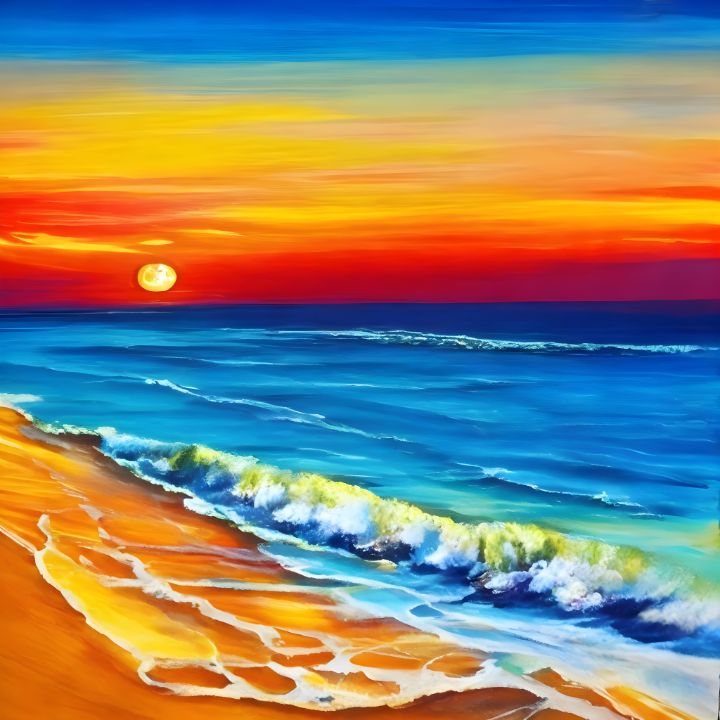The painting captures a serene seashore at sunset, presenting a vivid contrast of light and dark shades. The sky transitions from a deep red and orange near the horizon to a warm yellow, culminating in a tranquil blue higher up. The flat horizon hosts a glowing yellow sun, low in the sky amidst scattered clouds. Below, the majestic ocean transforms from a dark blue in the distance to a brighter hue in the foreground. White ripples from the waves animate the ocean's surface, crashing energetically onto the beach. The foam and washout create intricate patterns as waves retreat, leaving traces of bright orange and yellowish sand glistening beneath. The scene is mostly concentrated in the lower left, where the beach meets the ocean, offering a captivating blend of natural elements and colors.